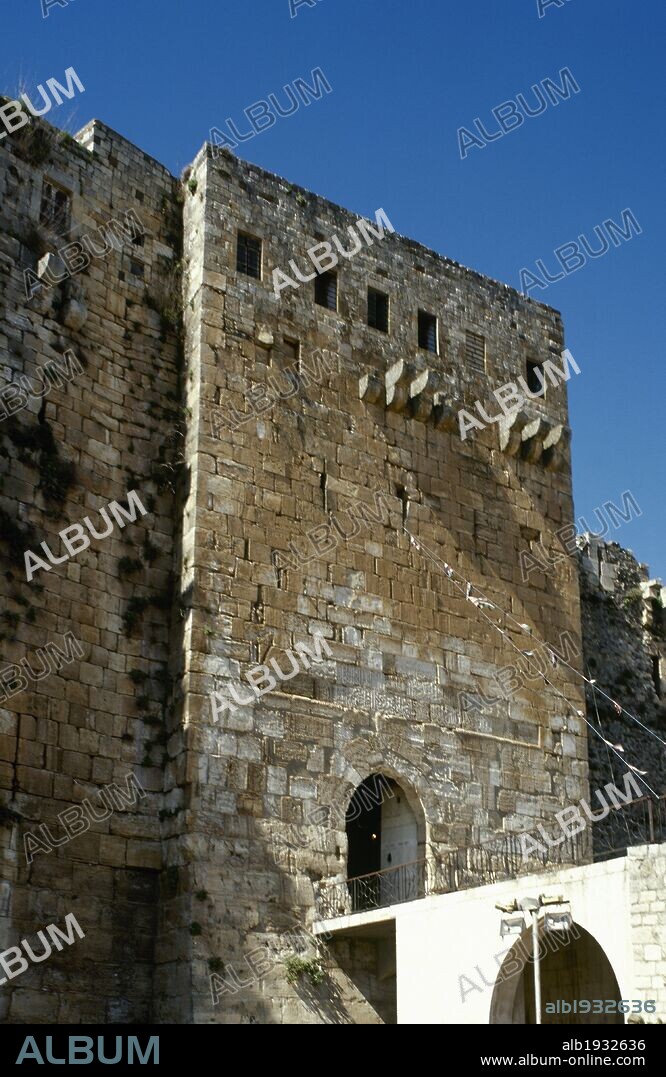The image features a historic, weather-worn stone wall reminiscent of a medieval castle with a distinctive bridge leading up to its entryway. The castle's brown stone bricks appear ancient and crumbling, contrasting with the newer addition of whiter bricks at the base. The structure boasts a rectangular front with high, narrow windows at the top, and additional sections on either side, both featuring similar windows. The sky above is a vivid, rich blue, adding a striking backdrop to the scene. Overlaying the entire image is a white, partially faded watermark with the word "album" printed diagonally multiple times, sometimes in solid letters and other times as outlines. At the bottom of the image, the code "ALB1932636" is visible alongside a URL, www.album-online.com, suggesting this may be an old vinyl record album cover.